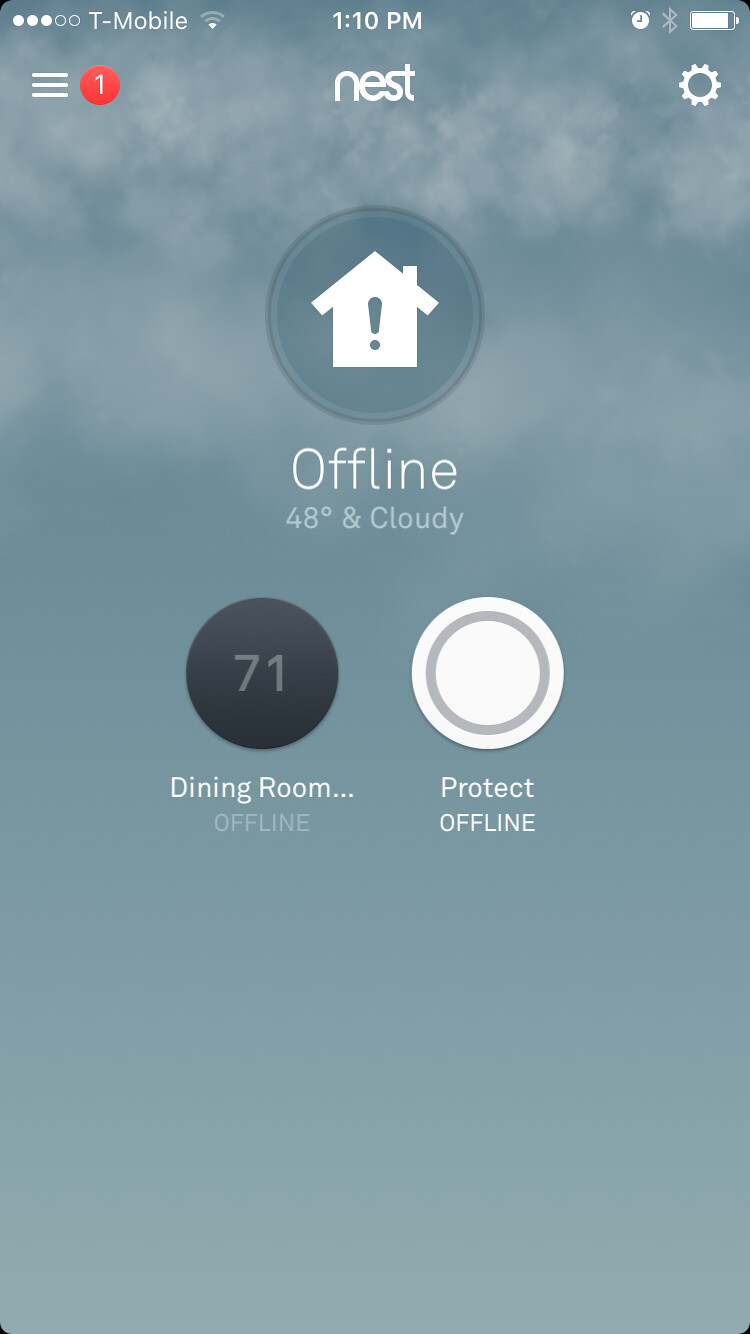The image displays the front screen of a cell phone. The status bar indicates the battery is fully charged, as shown by the battery icon, and the current time is 1:10 p.m. The status bar also shows connectivity information, including the word "NEST" and the carrier "T-Mobile." A three-line menu icon is visible next to a red circle containing a white interior.

The background of the screen features a clear blue sky with a few clouds. In the center, there's a large dark blue circle with a white house icon and an exclamation point inside it. Below this icon, the text "Offline" is displayed in white, alongside the temperature reading "48 degrees and cloudy."

Towards the lower section of the screen, a black circle with light gray text indicates the number "71" and underneath, it is labeled "Dining Room" in white text. At the bottom, there is a prominent white button with a silver circle inside it, featuring the text "Protect Offline" written in white.